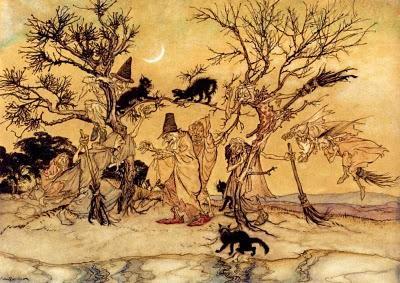The image is a detailed illustration with a distinctly Halloween theme, rectangular in shape and small, measuring about three inches wide by two inches tall. It depicts a chilling yet whimsical scene dominated by a group of raggedy old witches, each with a pointed hat and long noses, carrying or flying on their rickety brooms. The witches are gathered around two tall, barren trees, which are rendered in stark black hues, mimicking the eerie atmosphere of the illustration. 

Black cats, which are either perched on the branches or prowling on the ground, add to the spooky ambiance. Some cats appear to be meowing or fighting with each other, augmenting the noise and chaos of the scene. In the top center of the image, a crescent, silvery half-moon glimmers against a pale sky, enhancing the mystical feel. The entire illustration is bathed in shades of amber, yellow, gold, and tan, creating a vintage, aged effect. Given the subject matter and color scheme, this piece likely serves as an illustration for Halloween-themed content.